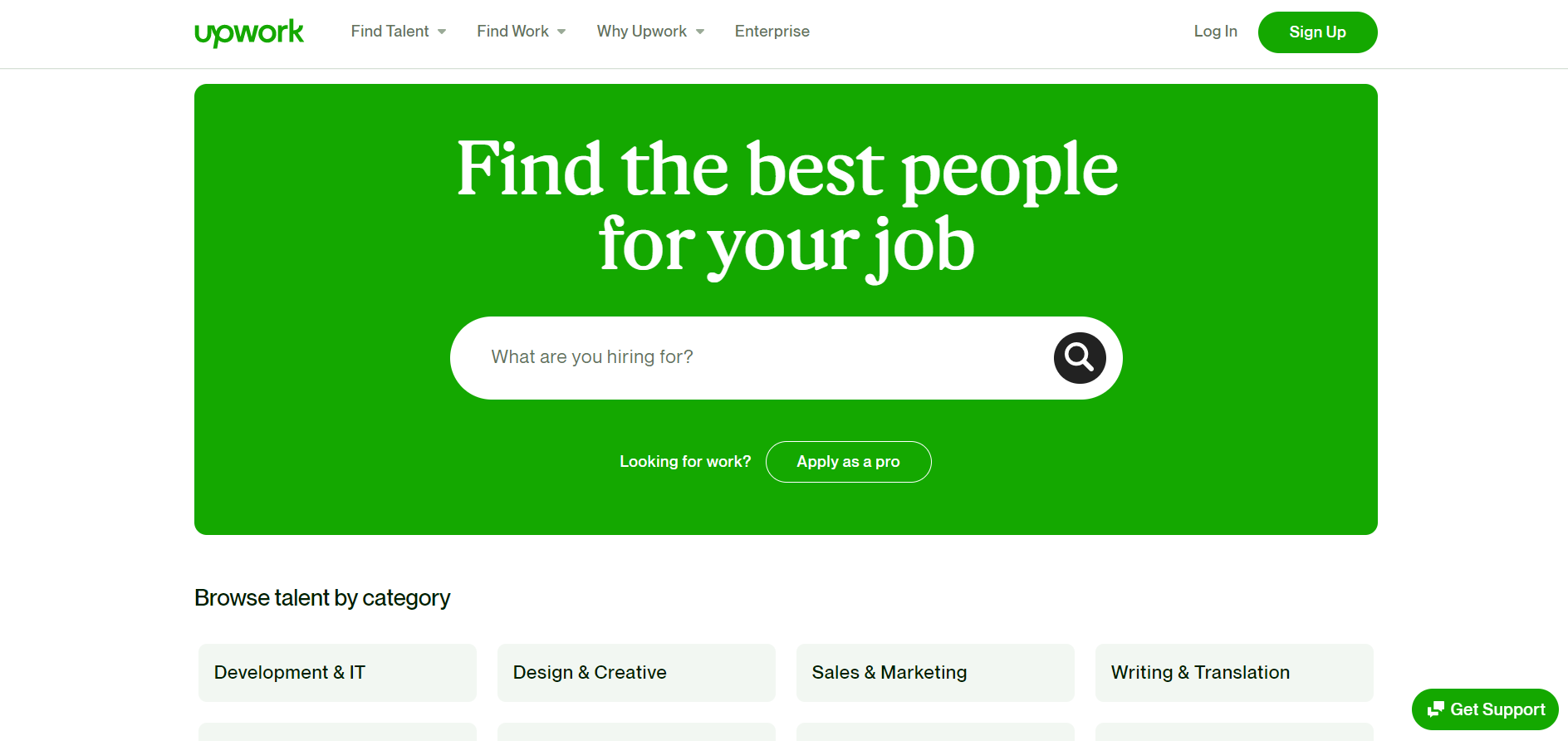The image features a clean, white background with a variety of UI elements from the Upwork website. 

In the top left corner, "Upwork" is written in green. To its right, sequentially in gray, are the text links: "Find Talent" with a drop-down menu, "Find Work" with another drop-down menu, "Why Upwork," which also has a drop-down menu, "Enterprise," and finally, "Log In." 

Next, towards the right, there is a prominent green, oblong-shaped button that says "Sign Up" in bold white letters. Below these elements extends a light gray line spanning the entire width of the image.

Beneath the line, a large green rectangle contains the text "Find the Best People for Your Job" in large, bold white letters. Below this rectangle, there is a search text box labeled "What Are You Hiring For?" with a black circle containing a magnifying glass icon. Additionally, there is a link saying "Looking for Work?" and next to it, a button labeled "Apply as a Pro."

Further down, against the white background, the text "Browse Talent by Category" is prominently displayed, followed by four category buttons: "Development & IT," "Design & Creative," "Sales & Marketing," and "Writing & Translation." To the right of these category buttons, a green box with white text in the middle reads "Get Support."